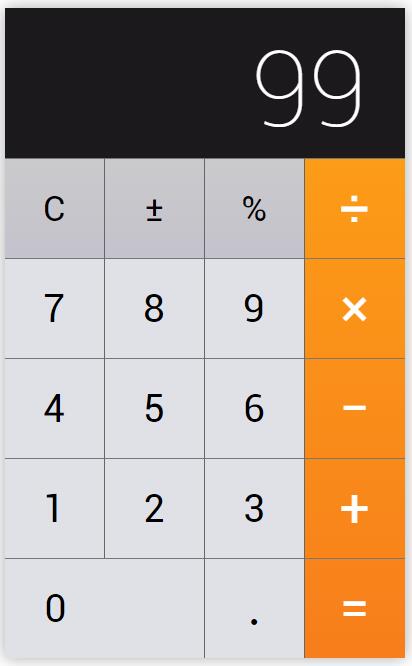This screenshot showcases the basic calculator interface of a smartphone. The main display at the top features the number "99" prominently in white against a stark black background. The calculator consists of a grid of buttons, organized by color and function: 14 grey buttons and 5 orange buttons. 

The grey buttons include number keys (0 through 9), a decimal point (.), and basic operations like percentage (%), a plus/minus toggle (±), and a 'C' button for clearing entries. 

The five orange buttons are reserved for key arithmetic operations: division (÷), multiplication (×), subtraction (−), addition (+), and the equals sign (=). The muted color scheme of grey and orange contrasts with the black and white display, lending a simple yet functional aesthetic to the interface. This is clearly a fundamental calculator app, intended for straightforward arithmetic without additional advanced features.